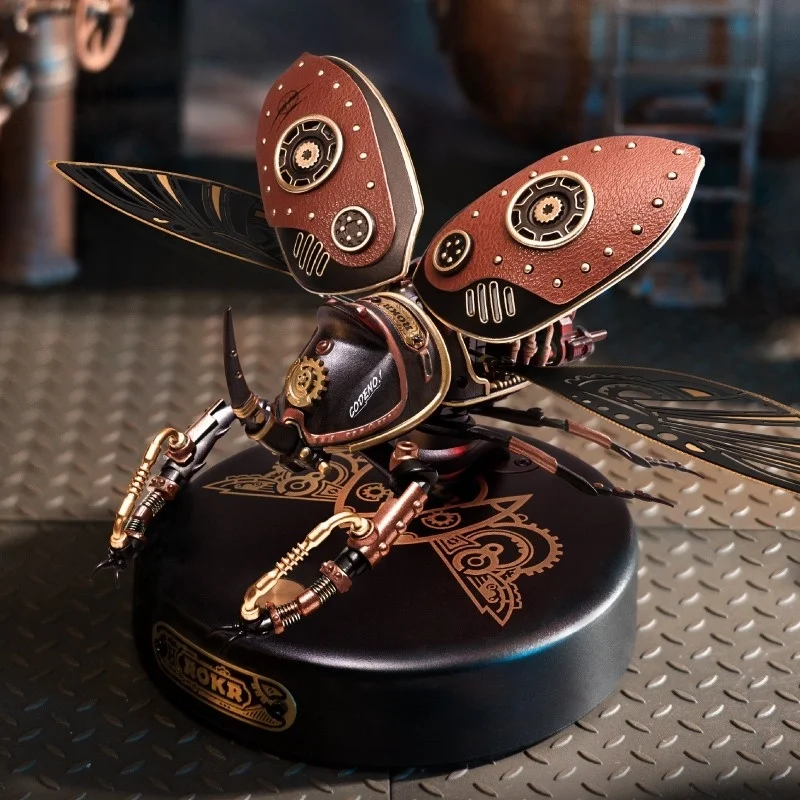The photograph showcases a striking 3D mechanical model of a beetle, meticulously crafted with intricate steampunk elements. The beetle, predominantly black with vibrant red and gold details, features prominent mechanical wings spread open, revealing gold detailing and rivets. It is equipped with large, metal pincers reminiscent of a crab's or scorpion’s claws, adding to its robotic allure. The model is mounted on a refined black and gold stand, inscribed with the letters "R-O-K-R" in elegant gold text and adorned with intricate design patterns. This setup rests on a textured surface that mimics metal but appears to be plastic. The background of the image is purposefully blurred, emphasizing the beetle, while faintly revealing an industrial setting with rusted pipes, a wheel, and other out-of-focus machinery. The high-quality image captures the essence of the mechanical insect, standing out vividly against its subdued, industrial backdrop.